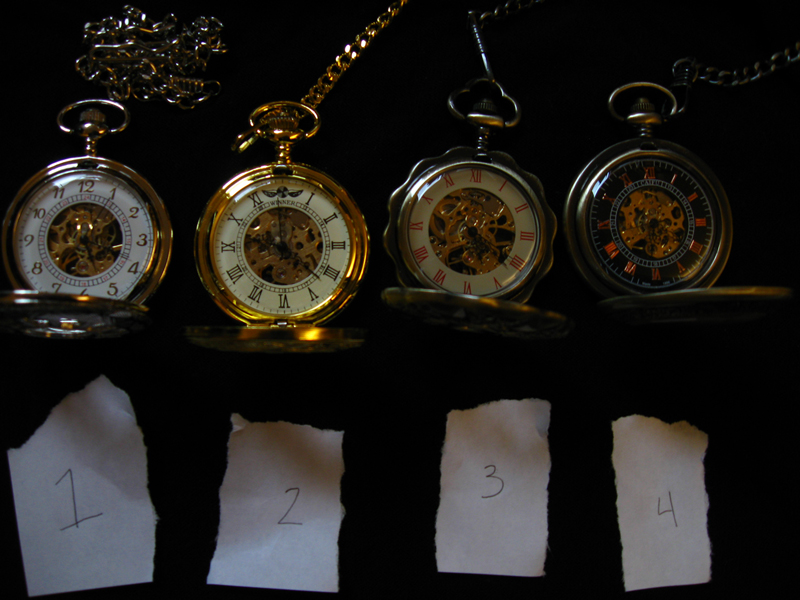This color photograph captures a dimly lit display of four pocket watches arranged in a row against a dark, possibly midnight blue background. Each pocket watch has a small chain attached to a loop at the top, exhibiting their traditional functionality. The first watch on the left features Arabic numerals, while the remaining three display Roman numerals in varying color schemes. The watches showcase a mix of materials—one gold, one silver, and two bronze—paired with white clock faces that highlight the numerals in black or red ink. Intricately designed, each watch reveals detailed craftsmanship, particularly in the center of the dials. Illuminated by light from above, this display case accentuates the contrast between the metallic watches and the dark background. Below each watch, a torn piece of white paper with numbers 1, 2, 3, and 4 serves as a reference, marking each timepiece’s position in the arrangement.